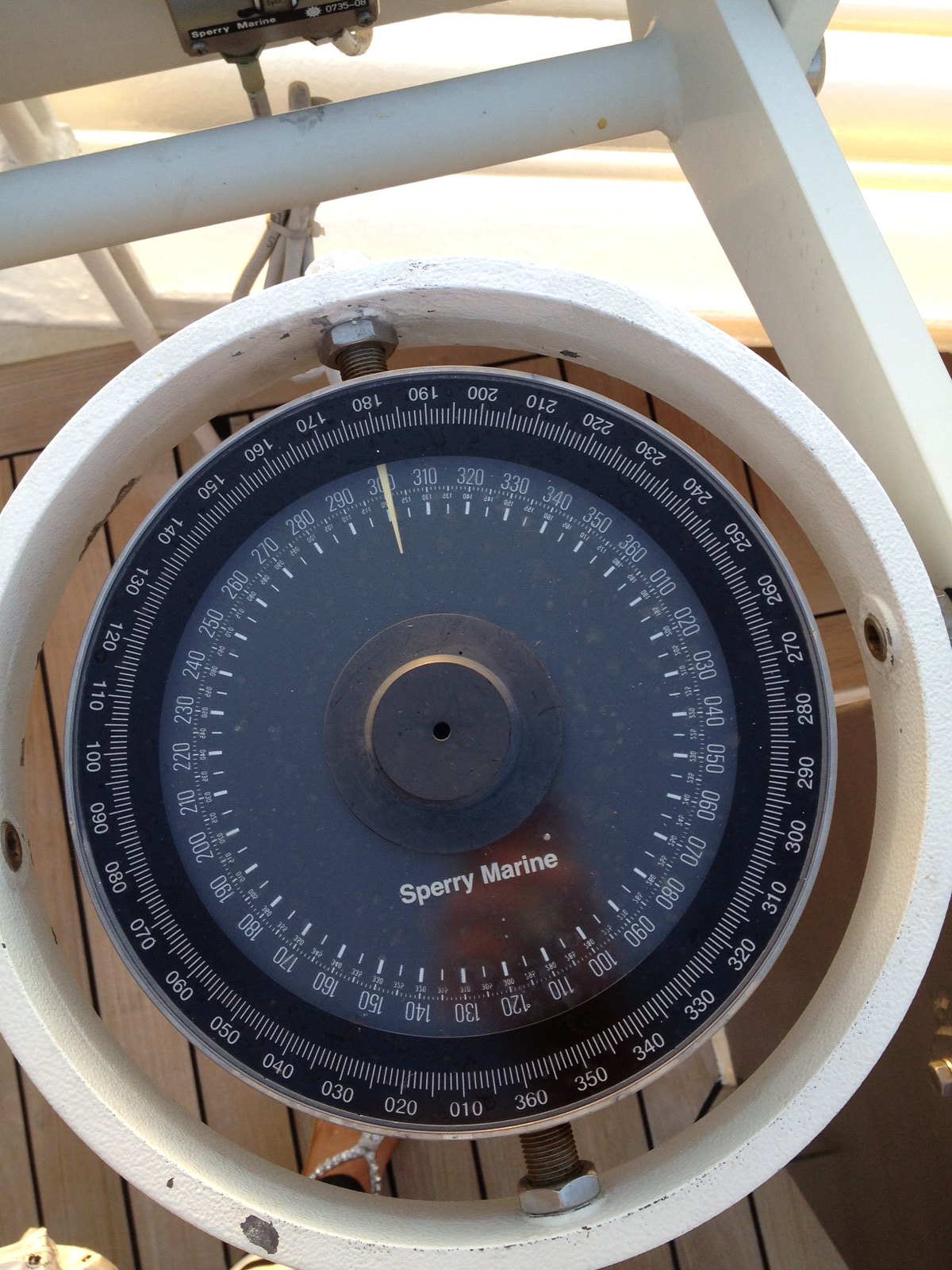A highly detailed caption for the image described could be:

"A close-up view of a precision maritime navigation device, securely mounted on a wooden platform. The device is encased within a sturdy, white, metallic housing, held together by four evenly spaced screws positioned at the cardinal points: North, East, South, and West. The screws at the North and South positions also fasten an internal circular component. The apparatus bears the name 'Sperry Marine,' indicating its maritime purpose. The outer rim of the device features a series of numerical markings, interspersed with fine vertical lines that form a complete ring. Nested within this outer circle is a secondary ring, also adorned with numbers and vertical lines, creating a layered and intricate design. At the very center lies another smaller circle, distinguished by a different material, featuring a central hole, potentially for calibration or reading purposes. The sophisticated design and detailed markings suggest the device is essential for precise measurement or navigation at sea."